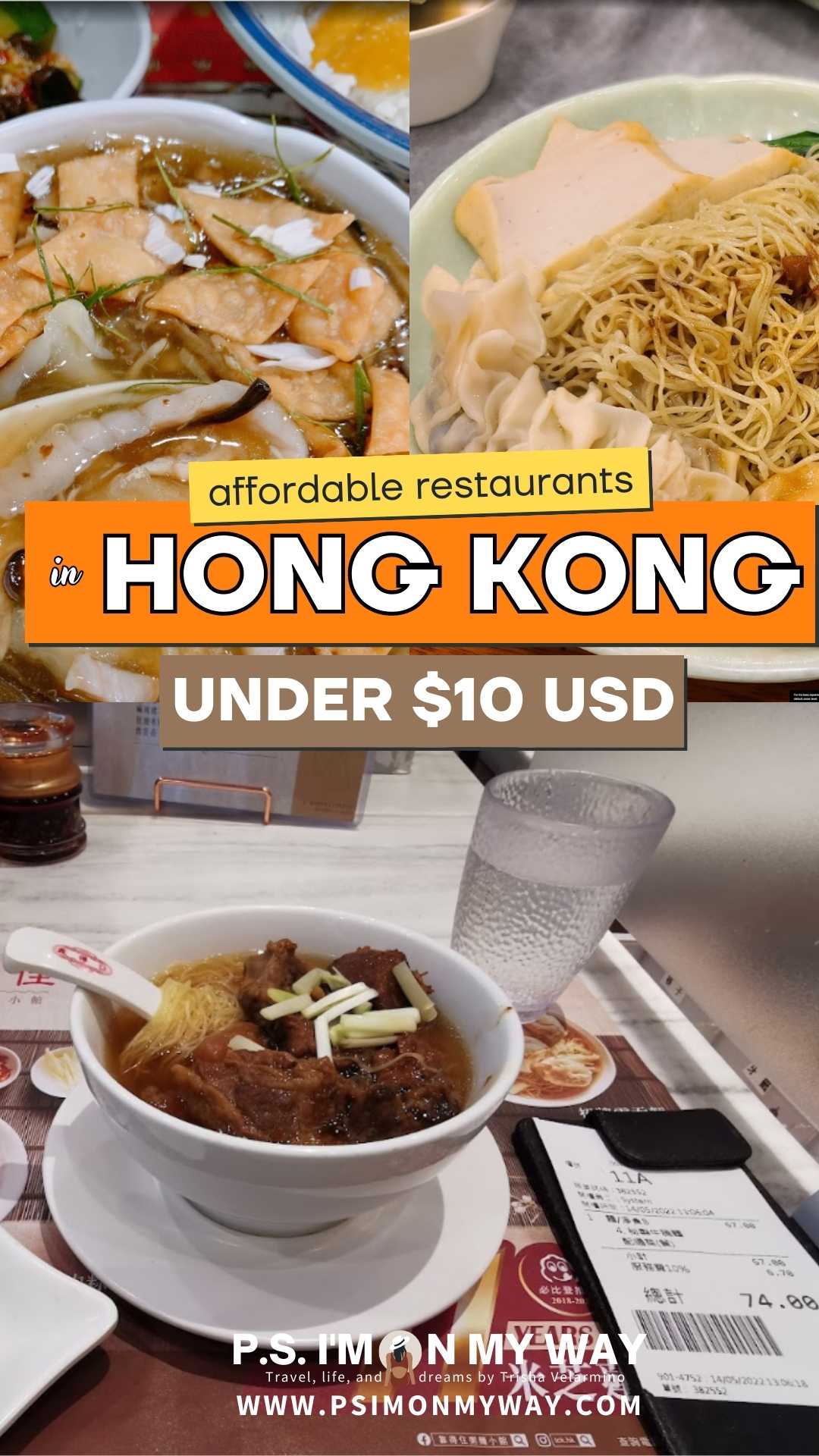The image is a flyer or website advertisement promoting affordable restaurants in Hong Kong where meals cost under $10 USD. At the center, there is text reading “Affordable Restaurants in Hong Kong Under $10” with each phrase highlighted in different colors: yellow, orange, and brown, respectively. Surrounding this text is a grid layout featuring three photographs of different dishes. 

In the upper left, there's a close-up photo displaying a flavorful soup with pasta-like dumplings, accented by an unidentified white ingredient. To the right, another image showcases a large dumpling filled with noodles, also in a soup or broth. At the bottom, a third image depicts yet another soup rich with noodles, accompanied by a glass of water and a bill noting 74 HKD. The visuals are vibrant with a mixture of colors including orange, light brown, yellow, black, tan, beige, gray, and hints of red, set against a visually appealing background that suggests a magazine or brochure style. The overall design emphasizes appetizing, budget-friendly dining options with real, enticing photographs.